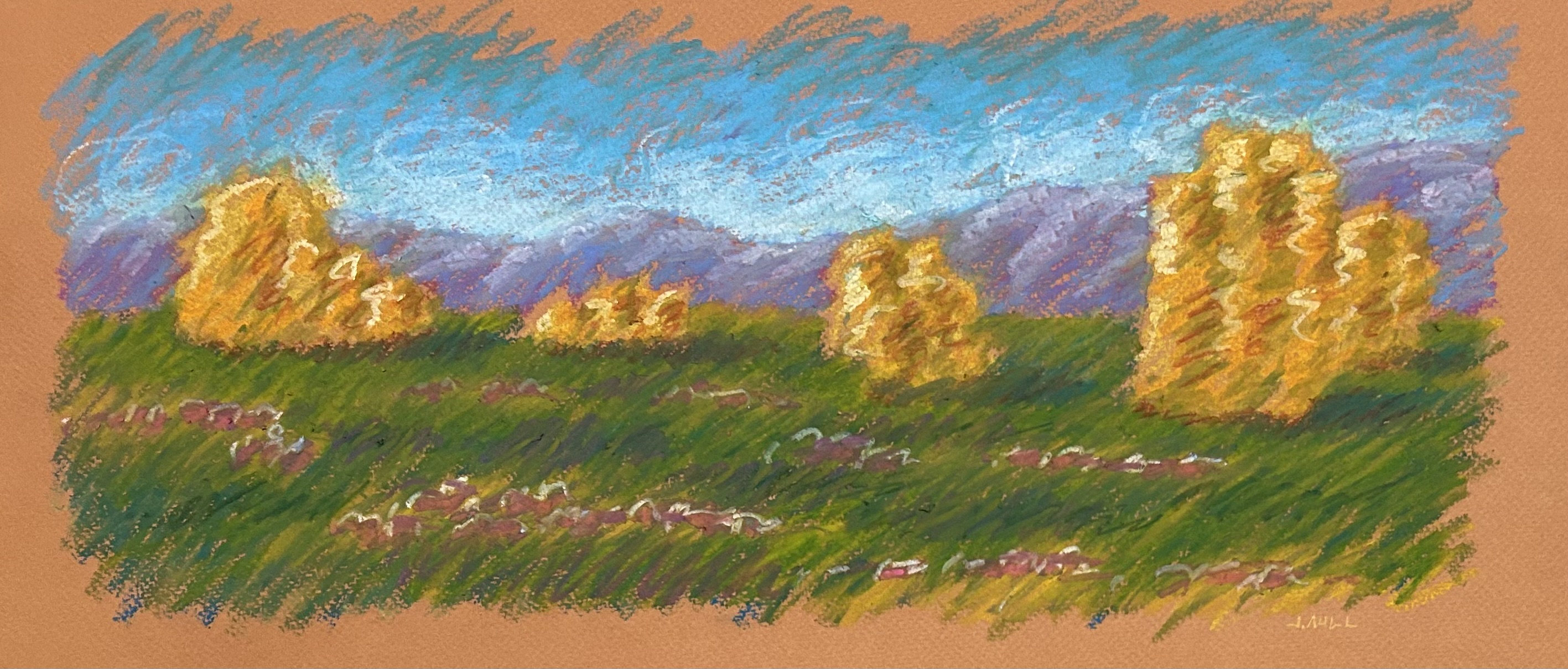This painting portrays a serene outdoor scene in an Impressionist style, characterized by vibrant and expressive use of color. The foreground showcases expansive fields of green grass interspersed with splashes of red and purple flowers. Prominently set against this verdant landscape are four golden yellow shapes that resemble either large groups of trees or haystacks. The background features distant purple mountains shadowed by a blue sky dotted with white clouds. The base of the painting has a peach or orange hue, possibly indicating the medium or background color used by the artist. The name inscribed on the right-hand side is partially legible, suggesting it might say "J-A-U-L-L." The overall texture and appearance suggest the use of pastel markers, contributing to the artwork's soft and dynamic aesthetic.